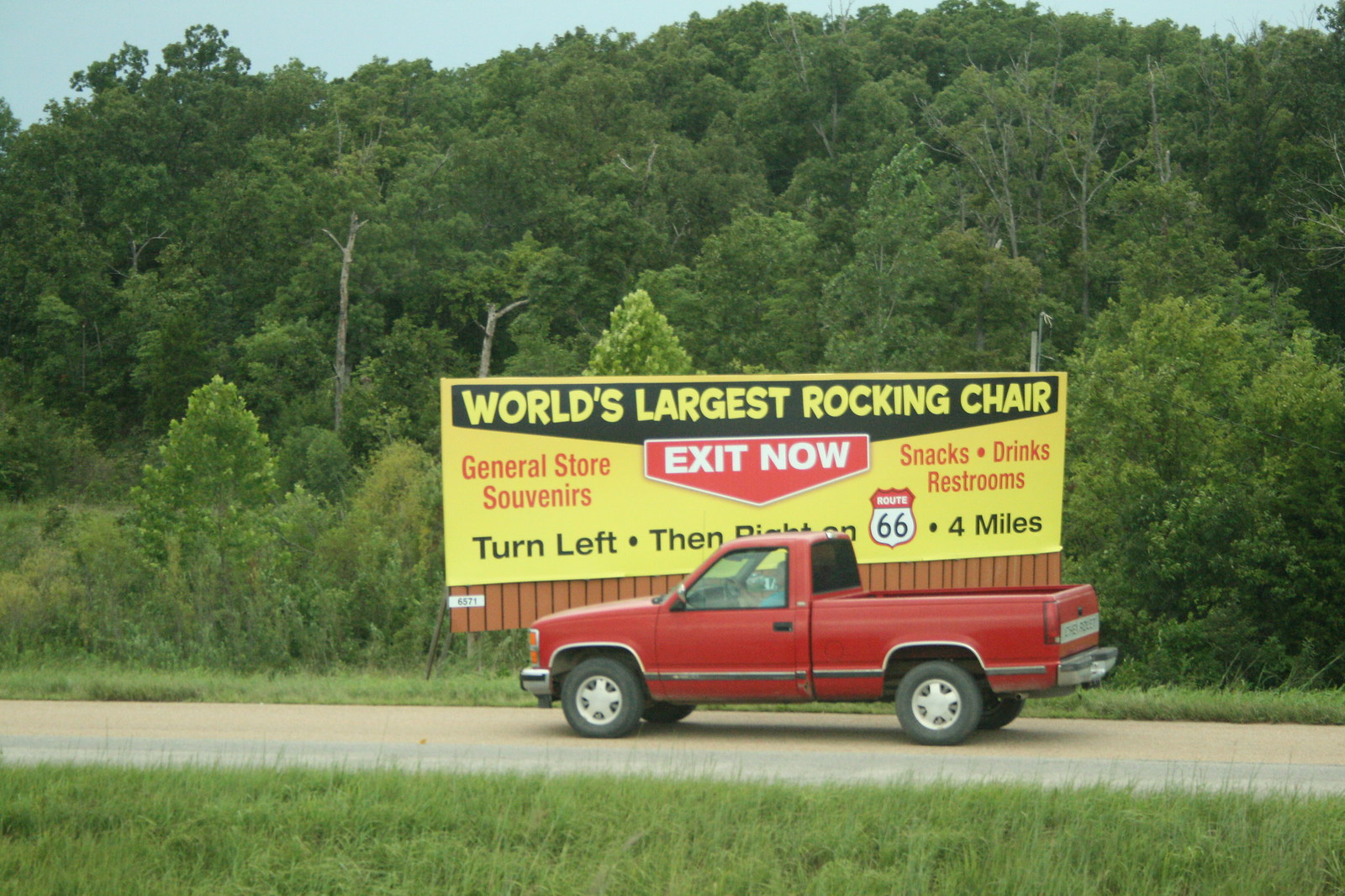In the foreground of this photograph, there is a patch of vibrant, lush green grass mixed with tall weeds. Just beyond this greenery lies a light gray, possibly paved road. On this road, an older, red Chevrolet truck is driving from the right to the left. The truck appears to be from the 1980s, with a person visible in the driver’s seat. Behind the truck, the area transitions into a sprawling backdrop of bright green trees and bushes that extend up a steep hill, completely concealing the ground beneath. The scene is set against a gently hazy blue sky that stretches above the treetops.

Prominently in the background, there is a large yellow billboard framed by a black border. The billboard announces in bold yellow letters, "World's Largest Rocking Chair," and features a red arrow pointing downward with the words "Exit Now." Below this, a red triangle contains white text detailing nearby amenities: "General Store, Souvenirs, Snacks, Drinks, Restrooms." Directions are provided: "Turn left then right on Route 66, four miles." The billboard itself is comprised of several wooden planks running vertically along the bottom, adding to its rustic appearance.